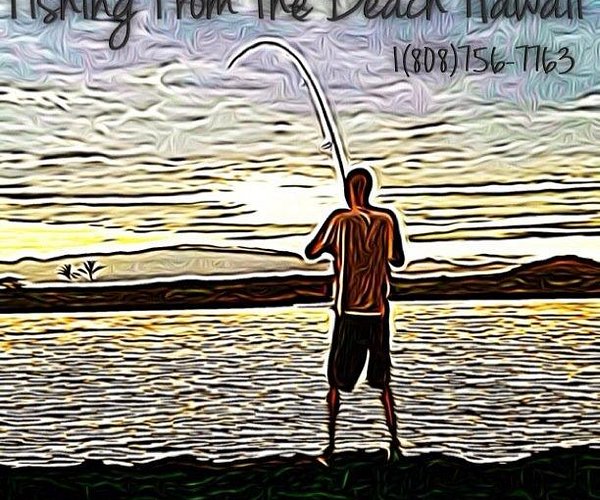The painting depicts a person, likely a man, fishing at the shore of a body of water, possibly in Hawaii, as suggested by partially visible text indicating "fishing from the beach Hawaii." The fisherman is positioned towards the middle-right of the image, standing on land facing the water, which shows ripples and extends towards a distant island with palm trees on the left. The scene features vibrant and contrasting colors including yellows, blues, grays, greens, blacks, and browns, suggestive of a sunset with the sky transitioning from yellow and orange near the horizon to blue and gray higher up. The man is characterized by a simple, slightly wobbly and dizzying effect with thin legs, wearing black shorts and having an orange upper body. His fishing rod curves upwards and to the left. There is text at the top of the image, partially cut off, in a slightly cursive style, accompanied by a phone number: 1-808-756-7763. The overall image has a filtered and wavy appearance, adding to its unique aesthetic.